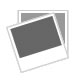The photograph features two wooden sculptures of elongated, stylized human figures displayed on a bright white table against a backdrop of polished brown wooden cabinets. The sculpture on the right depicts a very tall, thin woman wearing a knee-length dress that covers her arms. Her left hand is raised, appearing to balance a basket or jar on her head, while her feet dissolve into the wooden base. She is slightly leaning forward, giving a sense of movement.

The sculpture on the left represents a slender, headless male figure with an extremely long torso and arms. His left leg is bent at the knee and positioned forward, while his right leg merges into a large, narrow drum—resembling a bongo drum—that is placed between his legs. Both of his hands rest on the top of the drum. This figure is also elongated and appears to be naked, and, like the woman's sculpture, his feet dissolve into the wooden block.

Both sculptures exhibit detailed craftsmanship and are illuminated under bright lighting, suggesting an indoor setting, possibly an art exhibit or museum where traditional cultural pieces are displayed.